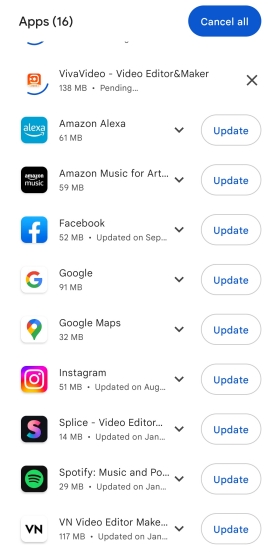The image appears to be a rectangular screenshot showcasing an app list. On the left side, the word "Apps" followed by the number "16" in parentheses indicates that there are 16 apps listed. On the right side, there's a dark blue rectangular button with white text that reads "Cancel All". The main portion of the image features a white background displaying the app list.

Each app entry includes a square-shaped icon on the left, followed by the app names written in black text. To the right of each app name, there are gray-outlined, almost rectangular buttons with rounded corners, displaying the word "Update" in blue text. 

The apps visible in the list include: 
- Amazon Alexa
- Amazon Music for Art
- Facebook
- Google
- Google Maps
- Instagram
- Splice
- Spotify
- VN Video Editor

Below each app name, the amount of space occupied by the app is shown, likely measured in megabytes (MB) or gigabytes (GB). Additionally, the date when each app was last updated is also displayed.